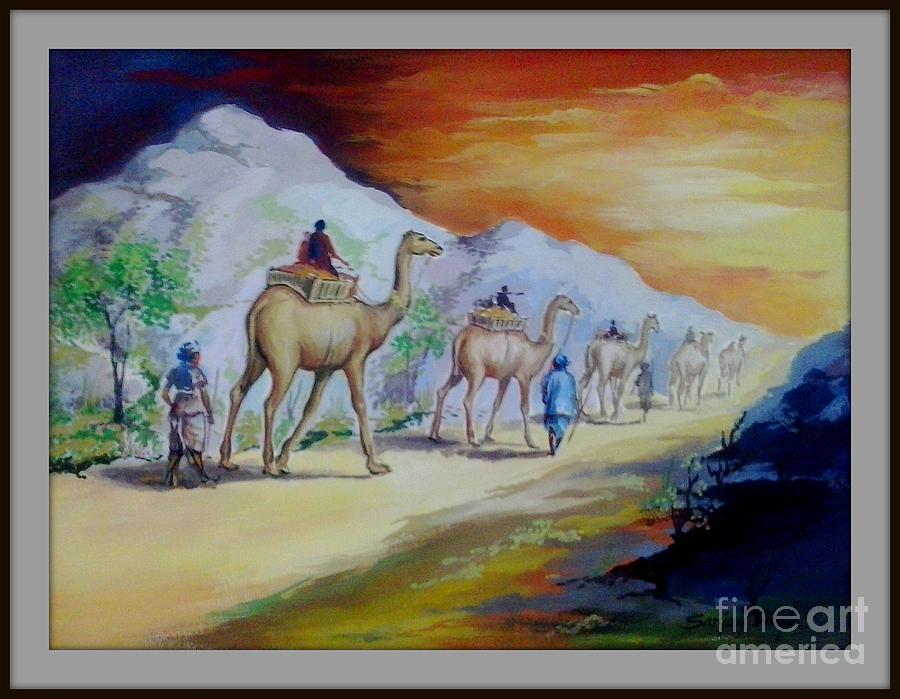This framed artwork, titled "Fine Art America" in the lower right corner, appears to be a print of an original watercolor painting, possibly depicting a Middle Eastern or North African scene. It features a camel caravan of five camels walking along a sandy dirt path during a vibrant sunset. The stunning sky transitions from a dark orange to a bright yellow, illuminating the landscape. The camels each carry a box-like structure, with one or two riders perched inside. At the back of the caravan, a woman follows behind the largest camel, which is guided by a man using reins. Two additional figures walk alongside the camels, assisting with sticks. To the right of the caravan, the path curves near blue-gray mountain outcroppings, while a lone tree stands sentinel to the very left of the scene. This serene image captures a slow, deliberate journey through an ancient, mountainous landscape.